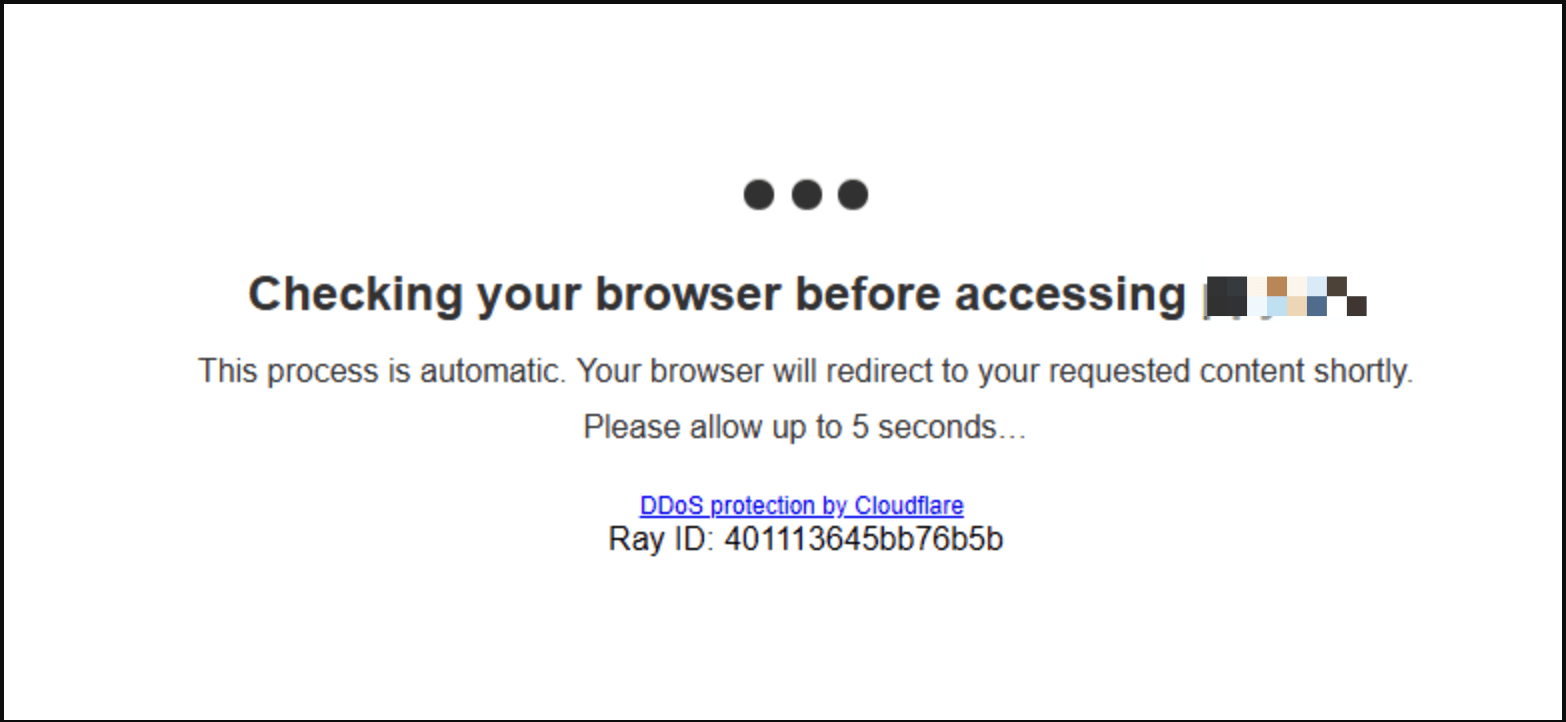An image captured from a computer screen displays a predominantly white background. Centered a few inches from the top are three black circles arranged horizontally. Below this, a message begins with "Checking your browser before accessing," followed by a section obscured by colorful squares and patterns, rendering the subsequent word unreadable. The text continues underneath in smaller font, stating "This process is automatic. Your browser will redirect to your requested content shortly." Further down, it instructs, "Please allow up to five seconds..." with an ellipsis.

Below this message is a noticeable blank space, followed by a clickable blue hyperlink in the center reading "DDOS_protection_by_Cloudflare." Lastly, at the bottom in plain text, it shows, "Ray ID: 401113645bb76b5b."